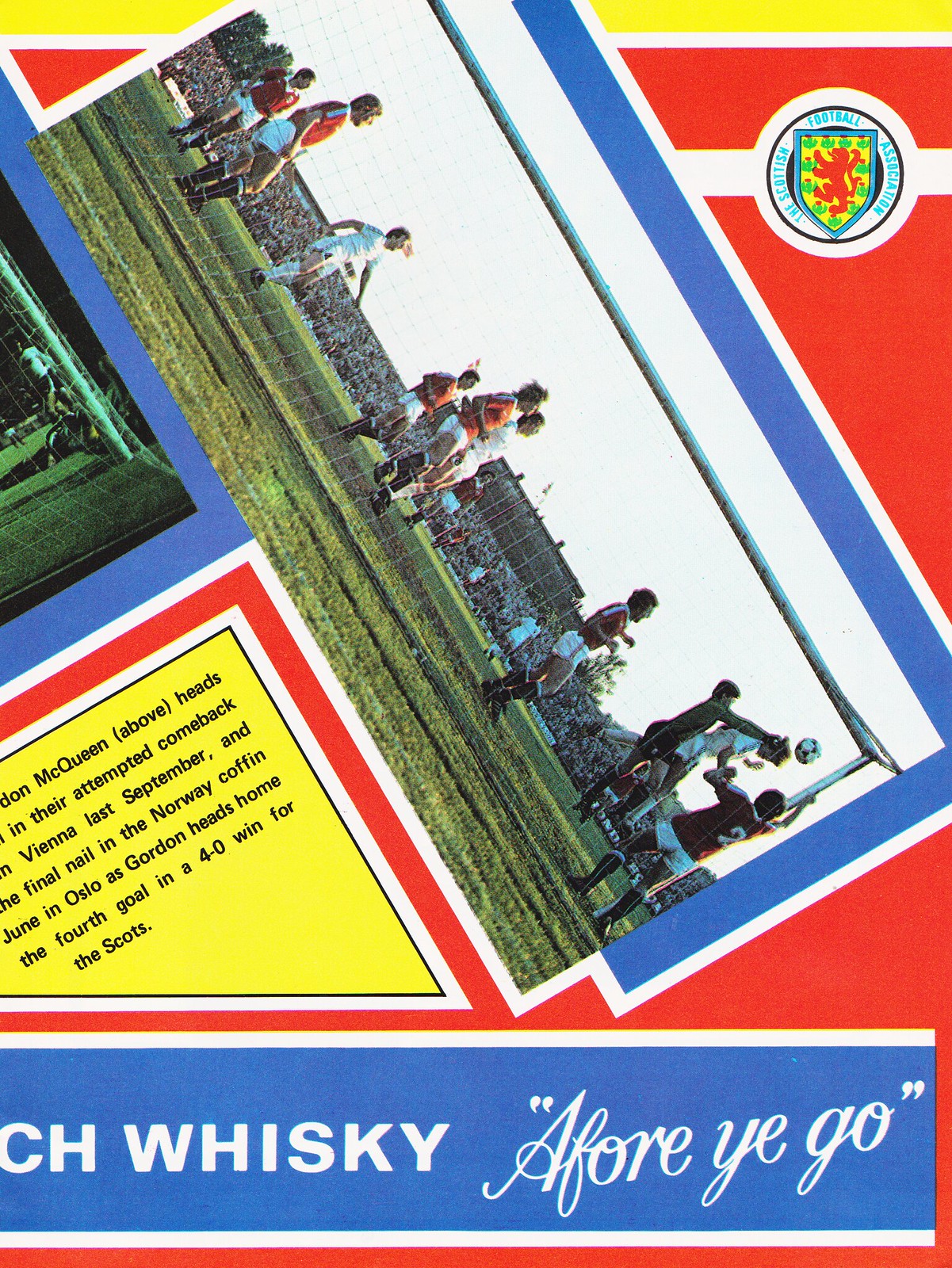This image appears to be a scanned page from a magazine or potentially a football club bulletin, likely tailored for a young audience, perhaps boys around 10 years old, to provide an accessible overview of the game and its players. The page features a vibrant red background and prominently displays the emblem of the Scottish Football Association in the upper right corner. This emblem, a heraldic shield with a red lion on a yellow field, suggests that the Scottish Football Association is presenting the content.

In the central part of the image, several blue boxes with white borders contain action photographs of soccer players during a match. These photos are arranged diagonally, creating a dynamic visual effect but making them somewhat challenging to view on a static monitor. The primary image captures a lively scene from a daytime soccer game, showcasing players in the midst of action on a crowded field with a packed stadium in the background.

Towards the bottom left corner, a yellow triangle featuring some text can be seen, but much of it is obscured by the image's boundaries, rendering it unreadable. Additionally, there is a partially visible word, followed by "whiskey" and the quote "a four year ago," suggesting an advertisement for Scotch whiskey along the bottom edge of the page. Overall, the page seems to serve as an engaging, visually rich piece aimed at discussing the sport, the players' skills, and perhaps promoting related products.